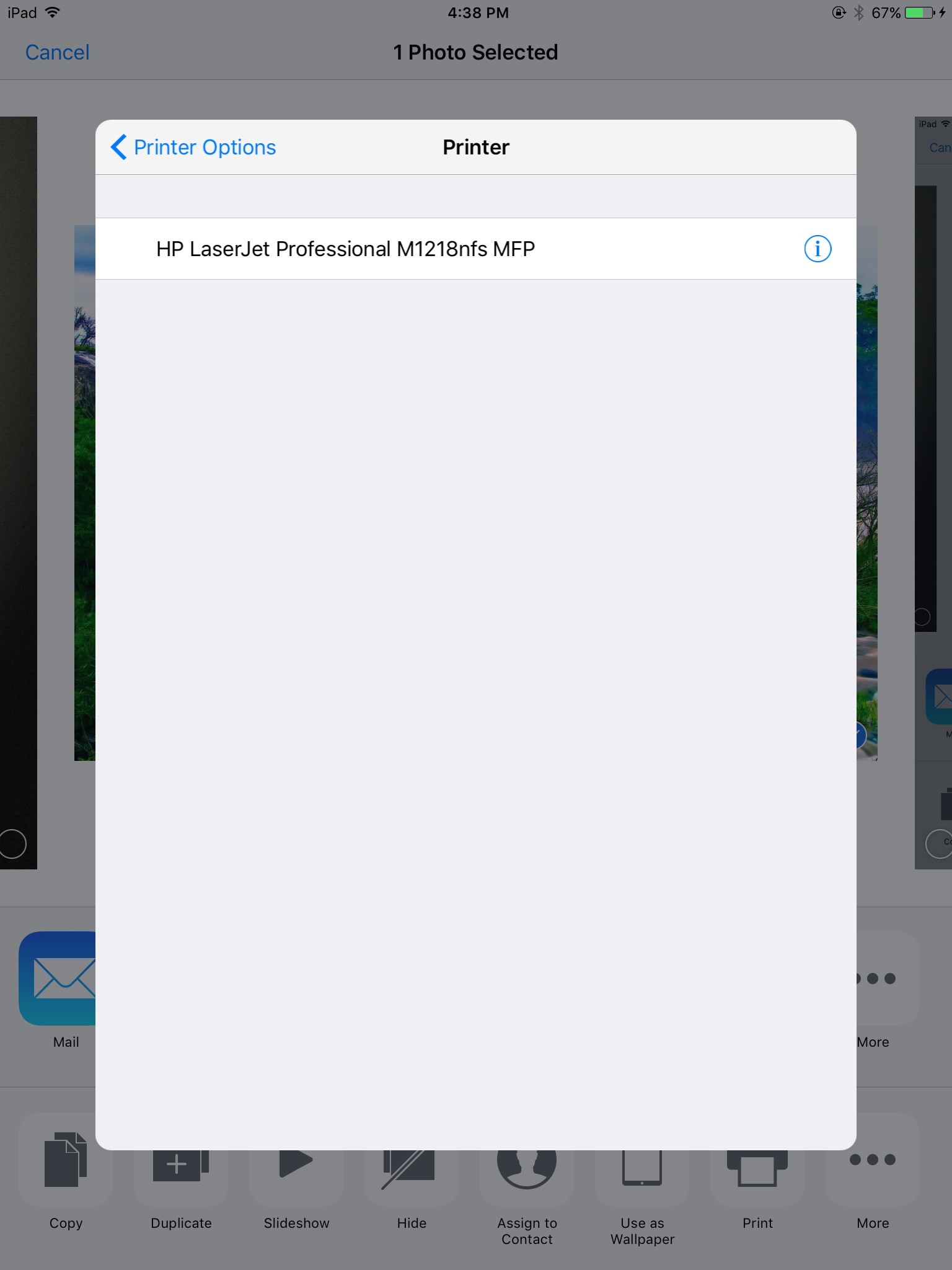A detailed screenshot depicting various options on an iPad screen. At the top, the status bar displays a battery icon at 67% with a thunder symbol indicating charging, alongside the time, 4:38 PM. The highlighted option is "Cancel" in blue. Below, there are multiple action options including "Copy," "Duplicate," "Slideshow," "Hide," "Assign to Contact," "Use as Wallpaper," "Print," and "More." 

Further down, a white square features "Printer Options" highlighted in blue, with a left-pointing arrow for navigation. Within this section, under the label "Printer," there is a white rectangle displaying the printer name "HP LaserJet Professional M1218nfs MFP" in all caps. To the right of this field, a blue circle with a blue lowercase "i" is present, likely indicating additional information or settings.